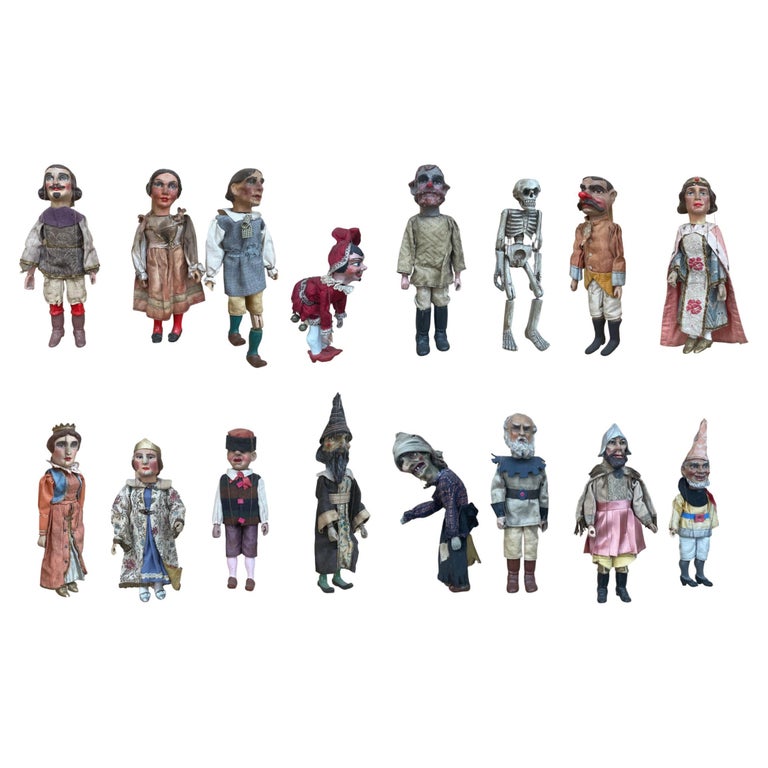This image features a collection of 16 distinct marionette figurines artfully arranged in two rows of eight against a white backdrop. Each figurine is meticulously detailed, reminiscent of an old-world setting, and a sense of timelessness permeates through their varied appearances. The top row showcases eight characters, including both men and women, some attired as old-time servants, while one stands out as a skeleton. Among these figures are individuals in period-appropriate clothing—intriguingly, one appears to be a ventriloquist doll blindfolded and without a hat. 

In the bottom row, the characters exhibit a richer diversity in roles and attire. Some figures don wizard hats, some represent royalty with crowns and silk-like robes, such as a queen in an oriental dress, suggesting a merging of cultural influences. A court jester in a red hat and jingling attire, gnome-like figures with pointy hats and large beards, and a figure resembling Pinocchio add to the eclectic assortment. There are mentions of shopkeepers and business people, adding everyday characters to the mix. This curated composition vividly captures a hodgepodge of different, uniquely shaped dolls with a vibrant narrative presence.